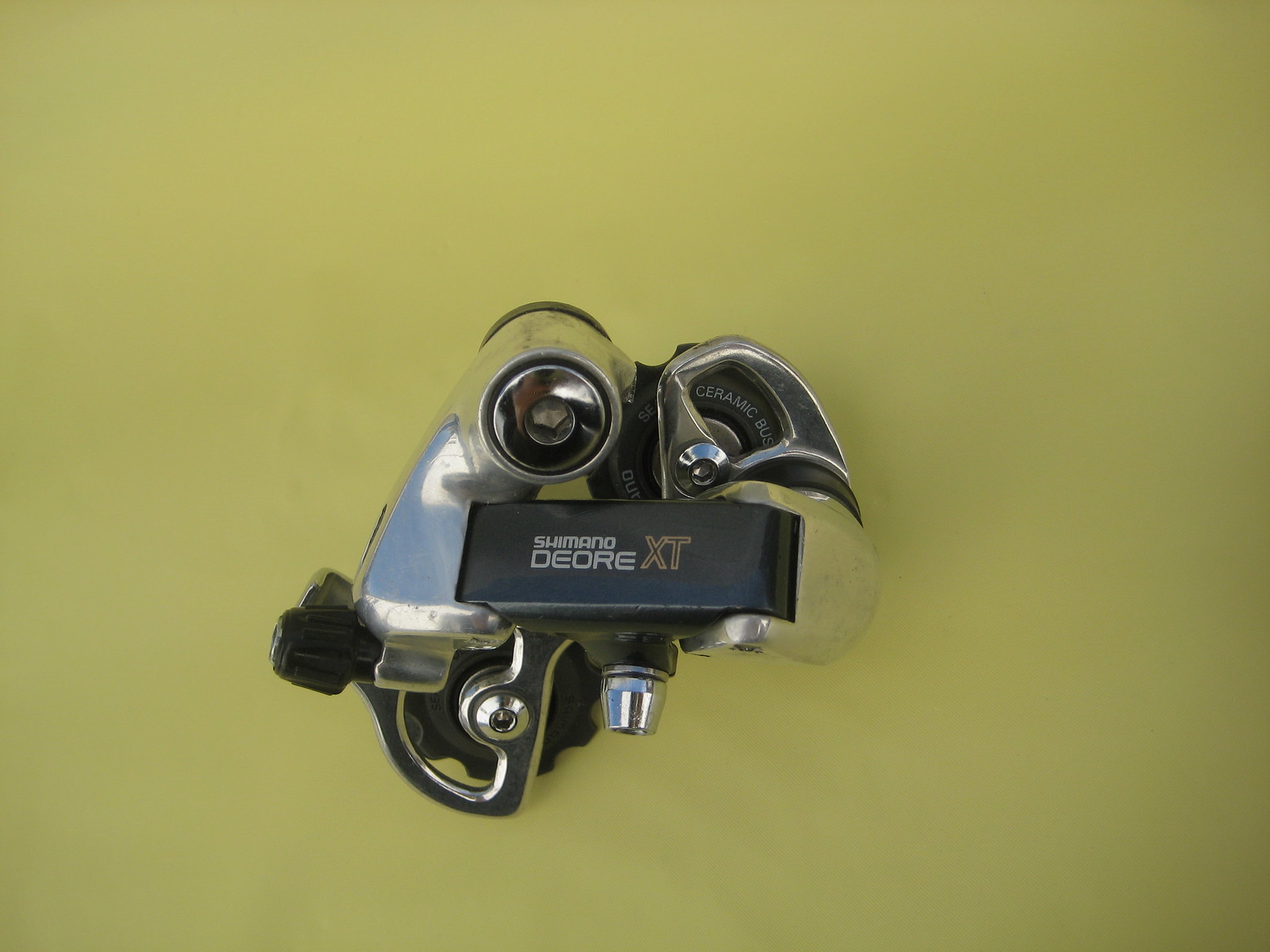This detailed rectangular image features a metal contraption set against a pea green background, centrally positioned but slightly lower in the frame. The contraption prominently displays a black plastic rectangular component with gray text reading "Shimano Diori" and adjacent brown text that reads "XT." On the left of this component, there is a silver metal object that curves outward and upward, culminating in a circular part. To the right, another curved metal portion connects to the first via a black plastic piece. At the bottom of the image, there is a visible black gear. The object is set in an indoor, staged environment, either mounted on a wall or lying flat on a surface, designed to highlight its intricate details and components.